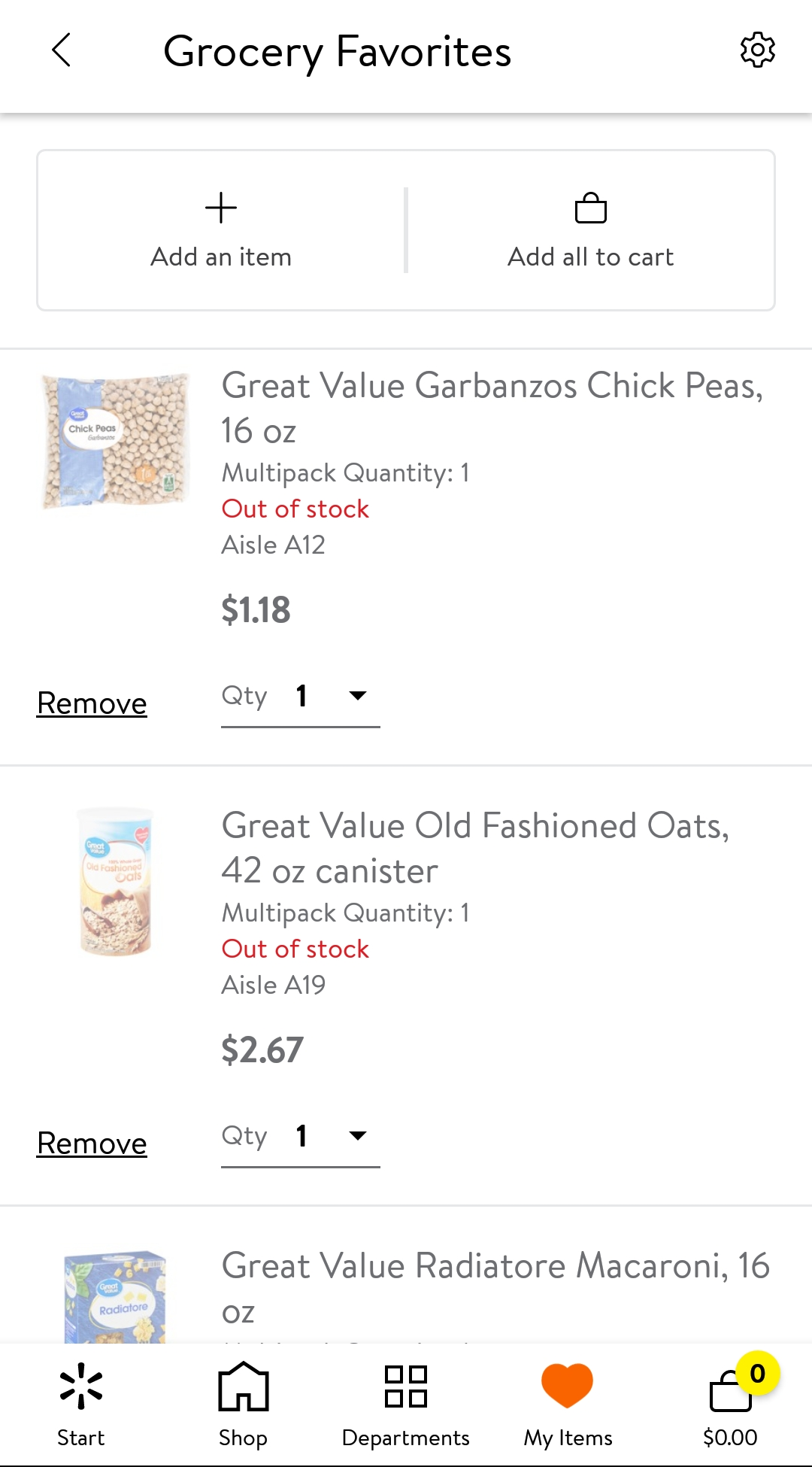The image displays a slightly blurry and compressed screenshot of a web page titled "Grocery Favorites" at the top center. Beneath this heading, on a white background, there are two buttons labeled "Add an Item" and "Add All to Cart," arranged from left to right.

1. The first featured item is "Great Value Garbanzo Chickpeas." To the left, there is an image of a bag of garbanzo beans. The item is listed as a 16-ounce package, with a quantity of 1 in a multi-pack. The chickpeas are noted as being out of stock and located in aisle A12. The price is $1.18. Directly beneath the item image, there is the option "Remove," and to the right, the quantity is noted as "1."

2. The second item is "Great Value Old-Fashioned Oats." To the left, an image of a 42-ounce canister of old-fashioned oats is displayed. This item has a quantity of 1 in a multi-pack, is also out of stock, and is located in aisle A19. The price for the oats is $2.67. Similar to the chickpeas, the word "Remove" appears below the item's image, and the quantity is listed as "1" to the right.

3. The third item listed is "Great Value Radiator Macaroni." On the left side, there is an image of a box of radiator macaroni pasta. Just beneath the macaroni's picture, the website offers navigation options "Start," "Shop," "Departments," "My Items," and the "Cart" display, arranged from left to right.

Overall, the screenshot provides a detailed view of selected grocery items that are currently out of stock, alongside their prices and aisle locations, within a user interface that includes options for managing the shopping cart and navigating the website.